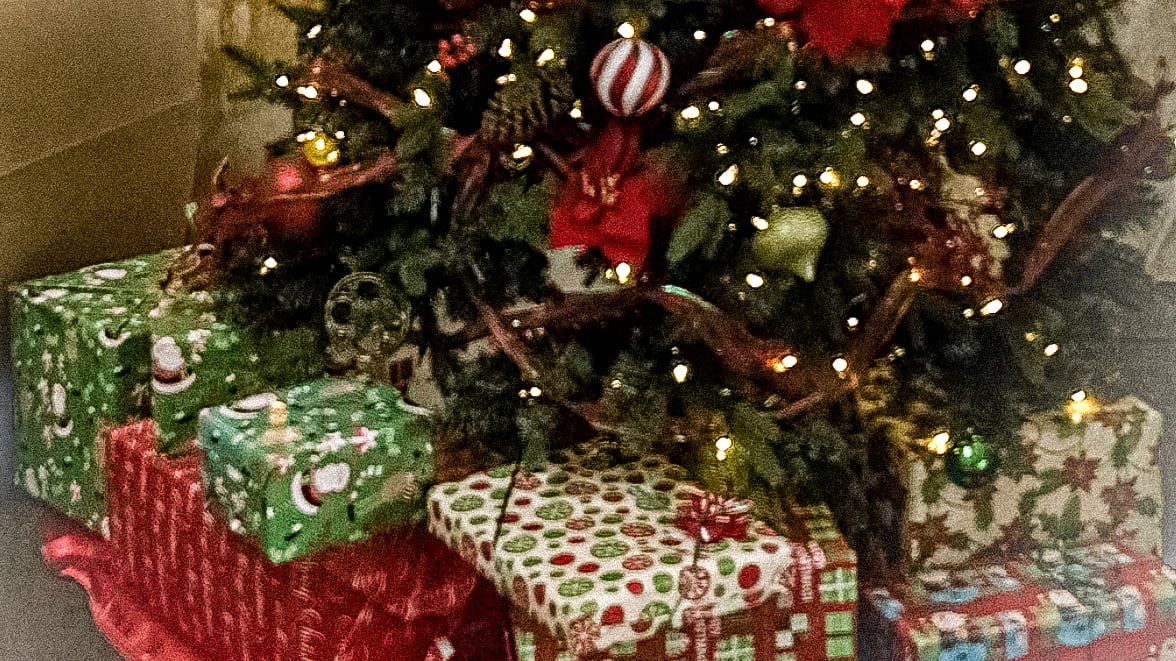The image captures a close-up view of the bottom third of an evergreen Christmas tree, adorned with a variety of festive decorations despite its slightly grainy quality. The tree is wrapped with dark ribbon and purple garland, and it glows with warm white lights scattered throughout its branches. Among the ornaments, there are red and white striped balls, green teardrop-shaped decorations, metallic-style ornaments, pine cones, and red flowers with layered petals. 

Beneath the tree, numerous presents are meticulously wrapped in assorted Christmas-themed papers. The packages vary in size and shape, ranging from large boxes to small, flat parcels. The wrapping paper features various designs: green paper with Santa Claus images, red paper with Christmas messages, white paper adorned with red and green balls, plaid red and green paper, white paper patterned with burgundy poinsettias, and even some blue and red designs. The close-up perspective highlights the festive atmosphere, focusing on the beautifully decorated tree and the colorful assortment of gifts below it.